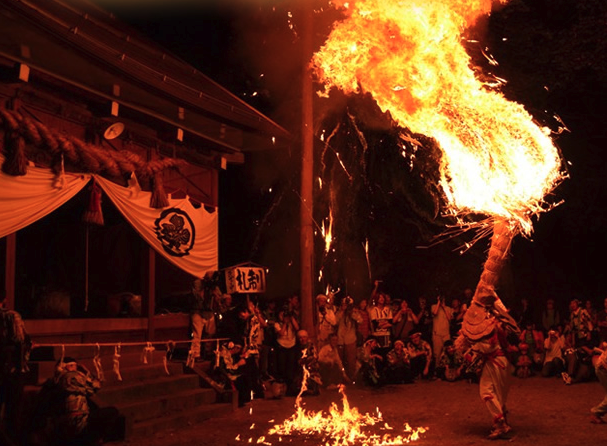In the image, a fire dance performance is taking place at nighttime, set against the backdrop of what appears to be a Japanese temple. The scene is illuminated only by the large flames coming from a pole held by a performer, creating a red hue that reflects off the surroundings. The fire is intense, engulfing the pole, and dripping molten flames onto the ground. A crowd of around 50 people is gathered at the back right, watching the performer intently. In the background, there is Japanese text on a pillar, adding an authentic cultural touch to the scene. To the left, a small, square shrine with a sloped roof and adorned with threads and floral prints stands, dimly lit by the firelight, accentuating the night’s darkness. The dirt ground adds to the rustic feel of the setting, emphasizing the traditional atmosphere of this captivating fire performance.